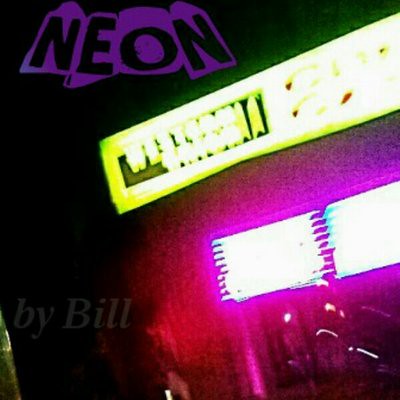In the image, the word "NEON" is prominently displayed in all capital letters, surrounded by a vibrant purple hue. A neon Western Union logo sign emerges from the top right corner, stretching diagonally across the image. The words "Western Union" are positioned on the far left end of the sign. Below the sign, two illuminated square-shaped lights, resembling grates, emit a bright glow. The strong illumination from these lights creates a fuzzy, blurred effect around their surroundings, casting a purple tint onto the backdrop, making other elements in the image indistinct.